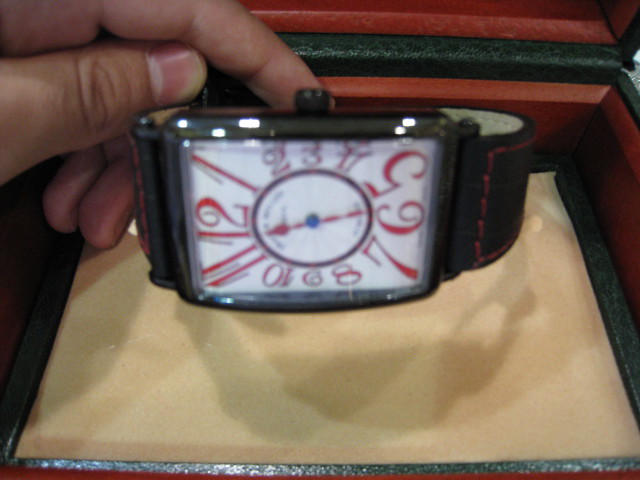A somewhat blurry close-up captures an elegant watch lying on its side atop a piece of soft beige fabric. The watch features a white rectangular face prominently displaying large red numerals. The number 12 is particularly striking in its size, along with the numerals 11, 1, 7, 6, and 5, while the remaining numbers are slightly smaller but equally vibrant in red. Matching red hands indicate that the time might be around 11:25:27. 

The watch is adorned with a black band that boasts red stitching along its edges, adding a touch of sophisticated contrast. A hand with slightly darker skin tone enters the frame from the left side, fingers positioned behind the back of the watch as though inspecting or adjusting it. The watch rests on the beige cloth, which appears to be part of a case lined with a striking combination of red and black material, enhancing the overall aesthetic and luxurious feel of the image.